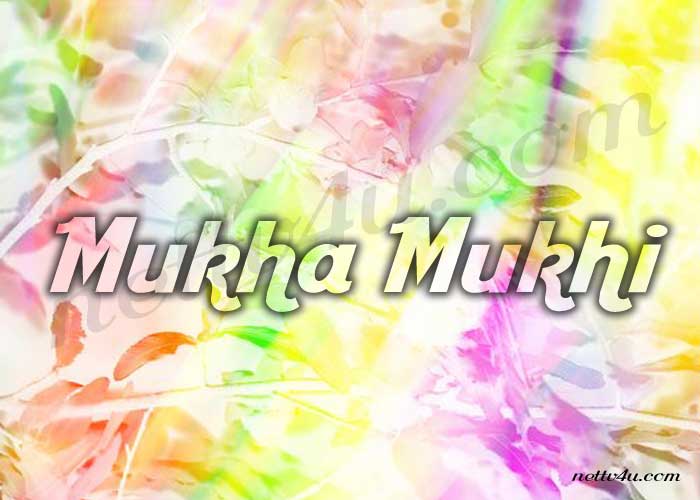This image bursts with vibrant and diverse colors, including purple, orange, green, yellow, and light blue, creating an artistic splash across the entire canvas. At the center, amidst the colorful background, is the text "MUKHA MUKHI" rendered in transparent font with a black outline. Reiterating its presence, the same website, "NETTVFU.COM," appears discreetly behind the main text. Additionally, in the bottom right corner, the website is clearly stated in black font. The overall effect is a vivid and dynamic composition, with a visually pleasing transparent window effect that highlights the central text.